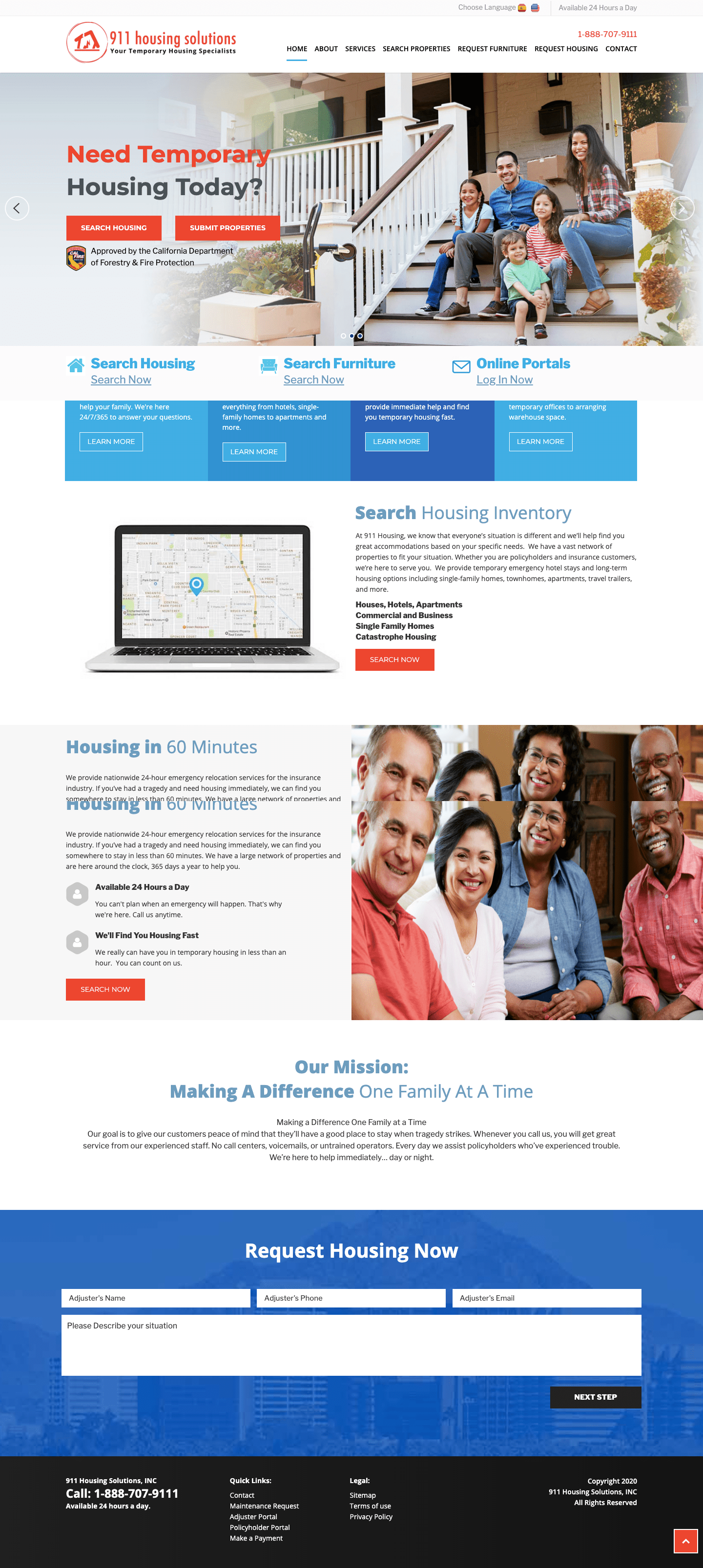In this image of a website, the layout is shown in a zoomed-out view, providing a comprehensive look at its structure and design.

Starting from the top left corner, there is the website's name and its prominently placed red logo. Adjacent to this, on the right side, is a small series of text in black, which seems to categorize different sections of the site.

Directly beneath this header area is a touching photograph featuring a family on their porch's staircase. The white railing frames the picture, which includes a mother, father, and their three children.

To the left of this family photo, striking red text reads "Need Temporary" followed by black text stating "Housing Today," accompanied by two bright orange rectangular buttons offering selectable options.

Further down the page, we see three distinct sections of light blue text, each featuring a name, followed by four blue squares below them. The third square is noticeably darker, and all squares contain selectable options.

On the left side, there's an image of a laptop screen, while to the right, the text "Search Housing Inventory" is displayed, followed by a paragraph of light black text and another orange rectangular button beneath it. Below this is a front-facing image of four individuals: a man in a red shirt, a woman in a white shirt, another woman in a blue jacket, and a man in a pink collared shirt.

To the immediate left of these individuals is a section providing additional information. Below this information, more details are displayed with blue text and black text following. An eye-catching blue rectangle at the bottom reads "Request Housing Now," accompanied by four fields for user input.

The website concludes with a bottom section painted in black, neatly wrapping up the visual layout.

Overall, the website's design balances text and images effectively, guiding the viewer's eyes through a logical flow of information while ensuring the crucial elements stand out clearly.